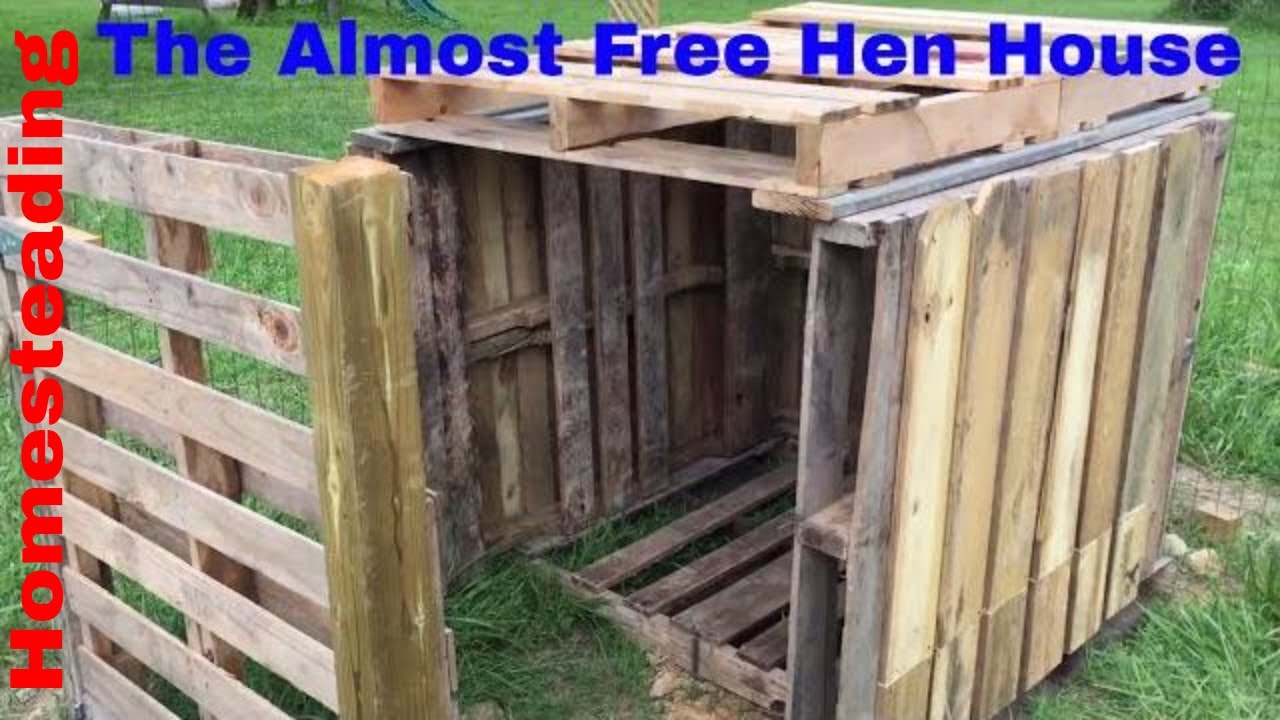This image features a makeshift hen house constructed from weather-worn shipping pallets, arranged to form a rectangular structure with four walls, a floor, and a roof. The coop is situated in the middle of a lush, green field, with long grass suggesting the presence of livestock. Text superimposed on the image includes the title "The Almost Free Hen House" at the top in blue font and "Homesteading" on the left side in red font. The overall impression is one of a DIY, resourceful project, utilizing repurposed materials to create a functional, though not particularly inviting, chicken coop.